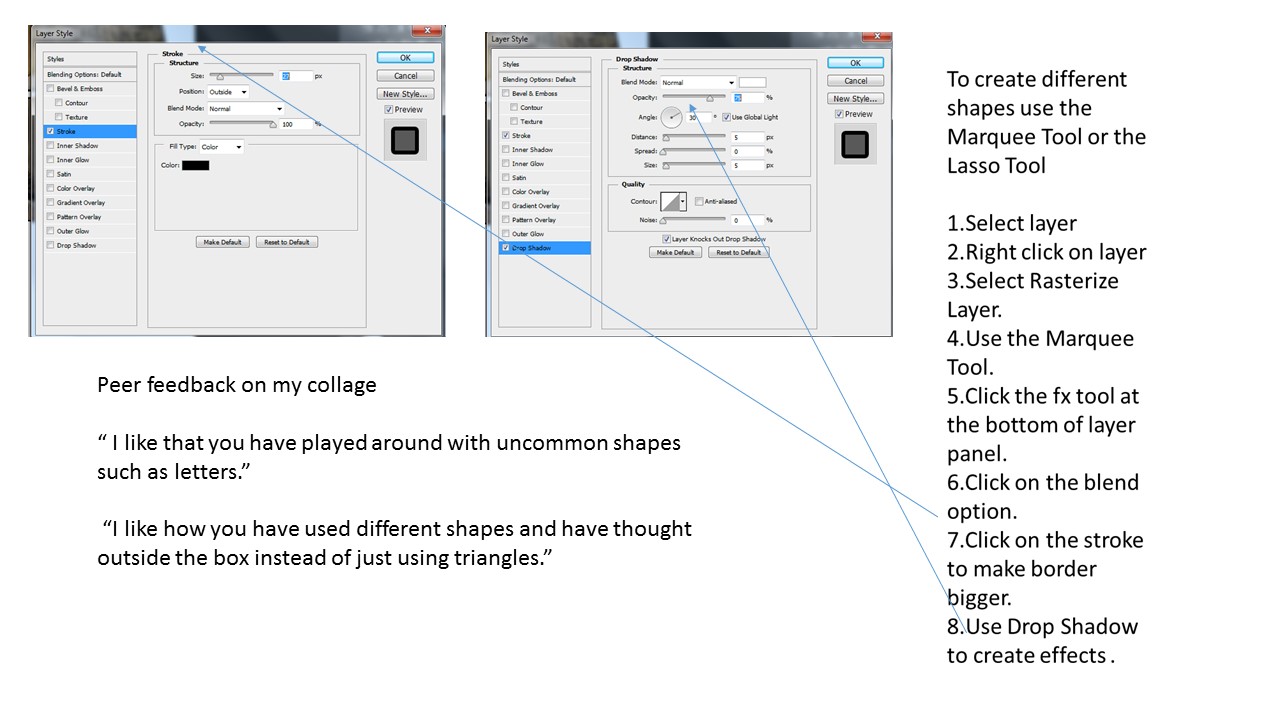The image depicts two gray Layer Style dialog boxes characteristic of a Windows operating system, each featuring various customization options like sliders and checkboxes for styling effects. The left-hand dialog box includes sections such as blending options, shadows, and structures, while the right-hand dialog box displays similar features. Both windows have the typical red X for closing, and buttons like OK, Cancel, New Style, and Preview, the latter of which is checkmarked. Above the dialog boxes is a white background with black text that reads, "Peer Feedback on my collage: I like that you have played around with uncommon shapes such as letters," and, "I like how you have used different shapes and have thought outside the box instead of just using triangles." On the right side, instructional text advises, "To Create Different Shapes, Use the Marquee Tool or the Lasso Tool," followed by a numbered list detailing steps for editing layers: (1) Select Layer, (2) Right-Click on Layer, (3) Select Rasterize Layer, (4) Use the Marquee Tool, (5) Click the FX Tool at the bottom of the layer panel, (6) Click on the Blend Option, (7) Click on the Stroke to make border bigger, and (8) Use Drop Shadow to create effects. Blue arrows connect the instructional steps to specific points in the dialog boxes, visually guiding through the process. The overall background of the image is white.